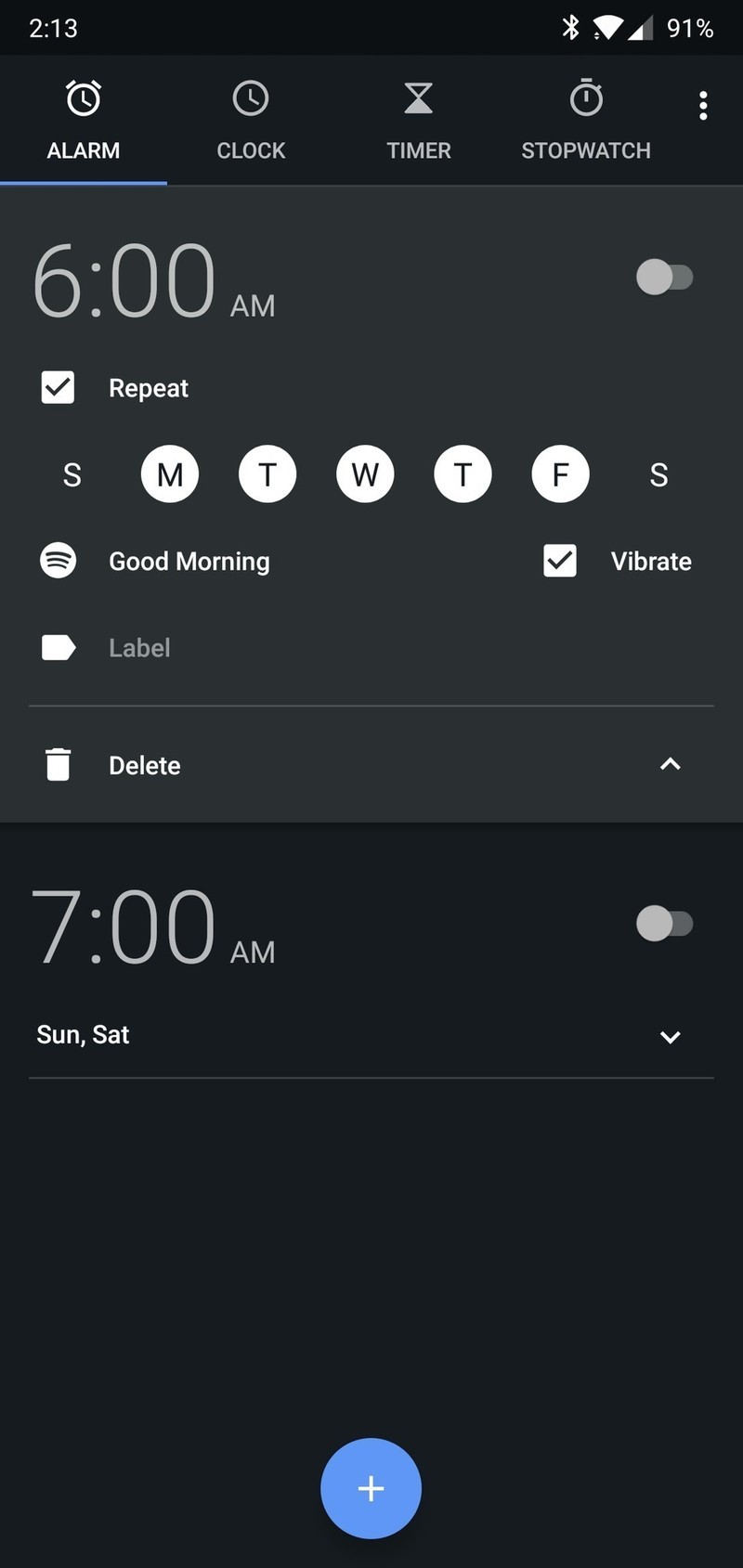The image showcases a black background interface, likely from a mobile device, displaying an alarm settings screen. 

In the top left corner, "213" is displayed in white font. To the right, a Wi-Fi icon is visible, followed by a signal strength chart, and a battery icon indicating a 91% charge. 

Below this, there are several icons and labels: 
- "Alarm" with an alarm clock icon above it
- "Clock" with a clock icon above it
- "Timer" with an hourglass icon above it
- "Stopwatch" with a stopwatch icon above it

A section highlighted with a blue underline indicates the "Alarm" is selected, with a gray line following beneath.

Below the icons:
- "6 a.m." is displayed in gray font on the left
- To the right, there is a small gray circle followed by a longer gray rectangle

Further down:
- On the left, a white square with a gray checkmark is labeled "Repeat" in white font
- Below this, a series of white circles with letters "S, M, T, W, T, F, S" indicate the days of the week, with Sunday marked twice, once at the beginning in a circle and once at the end in white font without a circle.

To the left, below a circle with three lines, the text "Good morning" appears.

On the far right:
- A white square with a black checkmark is labeled "Vibrate"
- Below that, a square with a triangular tip (an input field) is marked "Label." Underneath, a gray line separates an icon of a trash can and the text "Delete" next to a white arrow pointing right.

Further down, the text "7 a.m." appears in black font against the black background, accompanied by a gray circle to its right.

Underneath, "Sun, Sat" is written on the left, with a white arrow pointing down and a gray line beneath it.

At the bottom, a blue circle with a white plus sign in the center is present, indicating an option to add a new alarm.